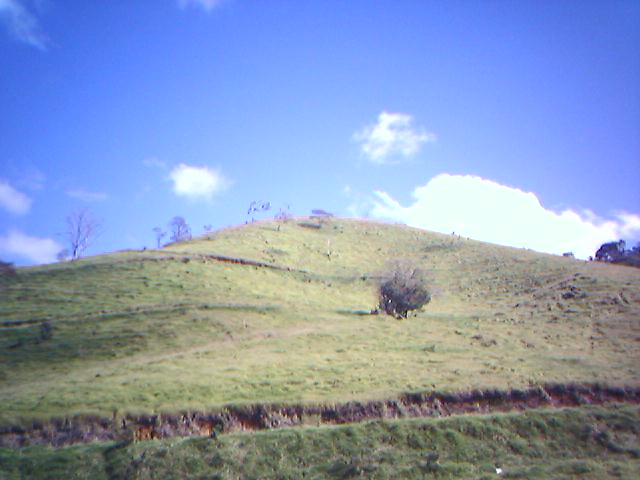This photo captures a serene outdoor scene featuring a grassy meadow that gently rolls up into a hill, which extends into a blue sky dotted with a few clouds. The foreground of the image shows a rut or path lined with taller, brownish grass or weeds at the base of the hill. The landscape includes a few small tiers as it ascends. On the middle and right third of the hill, there's a noticeable clump of small trees or tall bushes, adding a touch of greenery. The left side of the hill is sparsely populated with small trees that appear to be lacking in leaves. The sky above is mostly clear with some puffy clouds, including a prominent larger cloud in the right middle and a few smaller clouds on the left. This photo is bathed in natural daylight, highlighting the hill that dominates the center of the image, surrounded by blue, white, gray, green, brown, and tan hues.